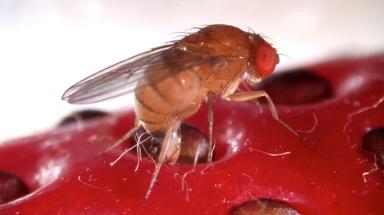The photograph captures a highly detailed, close-up image of a small insect, resembling a fruit fly, centered on a man-made surface. The insect's most prominent feature is its large, bright red eyes which dominate its head. Its body and thorax are orangey-brown in color, while its three visible sets of legs and two translucent gray wings stand out against the stark, bright white background. The insect is perched on a red, rubber-like material with multiple inset holes, giving the impression of a plastic surface or the bumpy texture of a fruit like a strawberry. The fly’s legs and thorax dangle over one of these holes, emphasizing the intricate details of the scene.